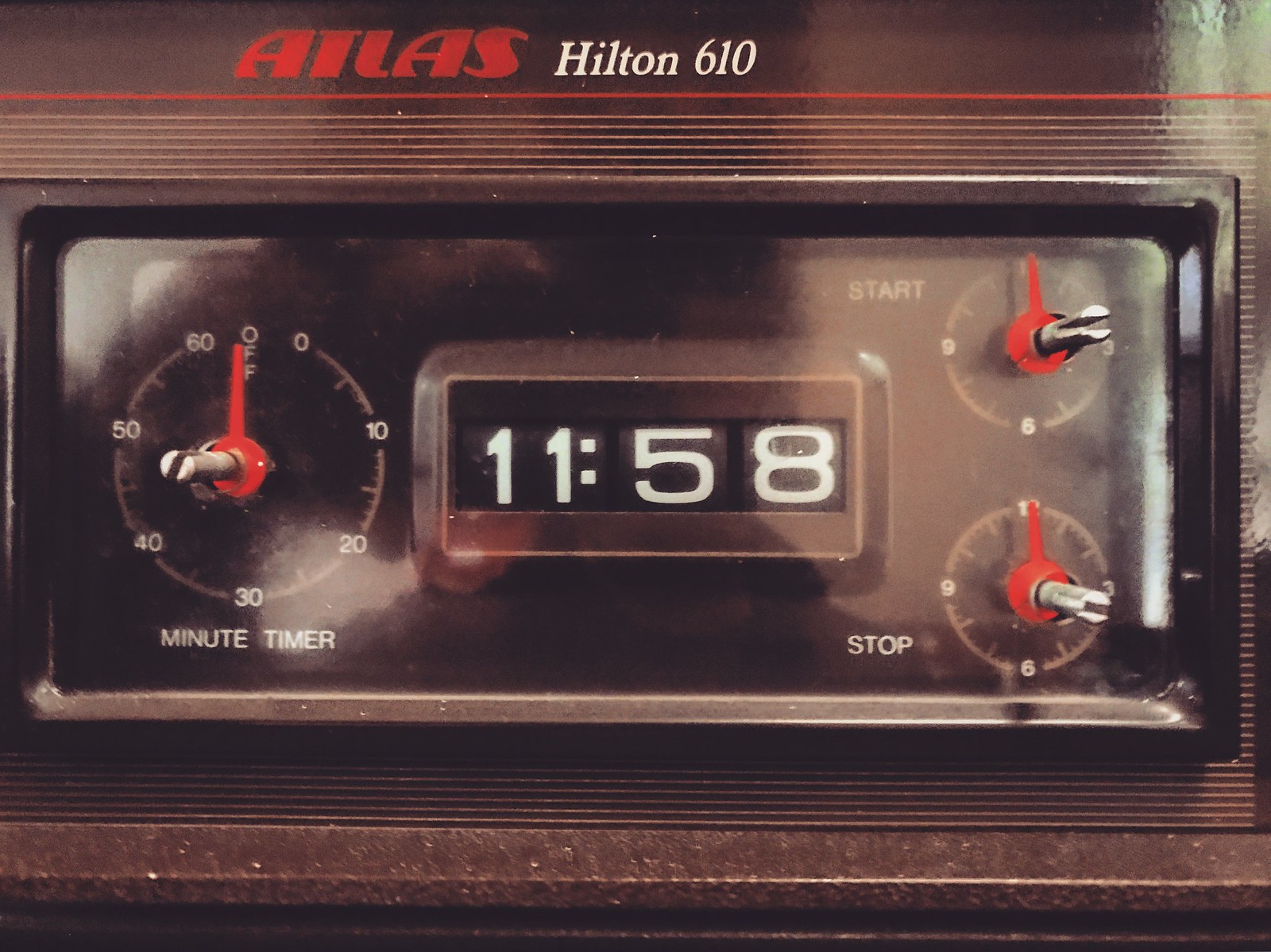The image showcases a vintage black device, likely a clock radio or an old Walkman. At the top, "A-T-L-A-S" is prominently displayed in red lettering, while below it, "Hilton 610" is written in white. Underneath this, a red line separates the branded text from a series of white lines, which add to the retro aesthetic of the device. Further down, a clear section reveals the time "11:58". To the left of the time display, there is a minute timer encircled with numerical indicators. On the right side, there are buttons labeled "Start" and "Stop", with corresponding controls for each function. Below this control area, additional white lines run across the device's surface. The entire design embodies a nostalgic, simplistic elegance typical of older electronic gadgets.